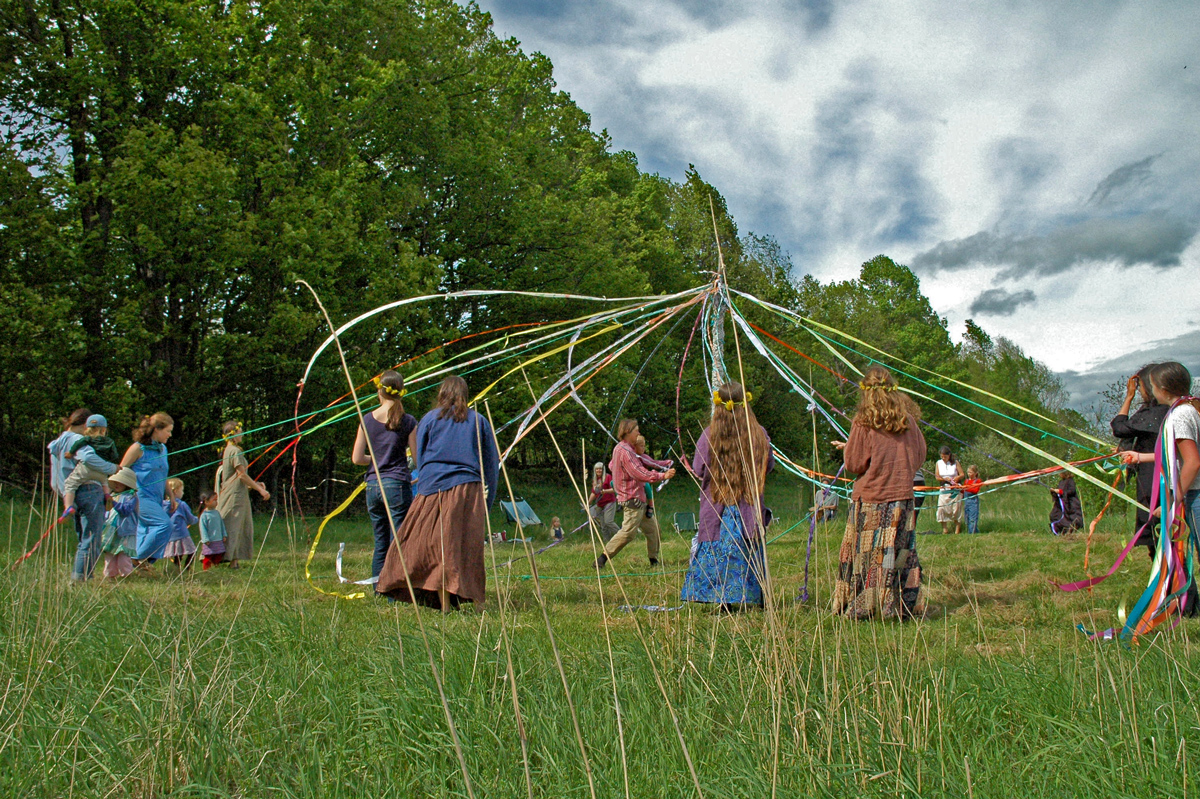The image captures a lively May Day celebration in a lush, green field bordered by tall trees. Central to the scene is a Maypole adorned with vibrant ribbons in shades of pink, blue, green, yellow, white, red, orange, and purple. About one and a half dozen participants, predominantly women and children, form a circle around the pole, each holding a ribbon. They appear to be dancing, wrapping the ribbons around the pole in a traditional manner. The women are dressed in flowing skirts and bohemian-style outfits, some adorned with yellow flower crowns, while children wear colorful clothing. A man stands in the middle, carrying a child, emphasizing the event's family-friendly nature. The background features a mix of dense green trees and a sky filled with fluffy white and gray clouds, underlining the casual and natural setting of this folkloric event. The overall feel is joyous and informal, capturing a moment of communal celebration.